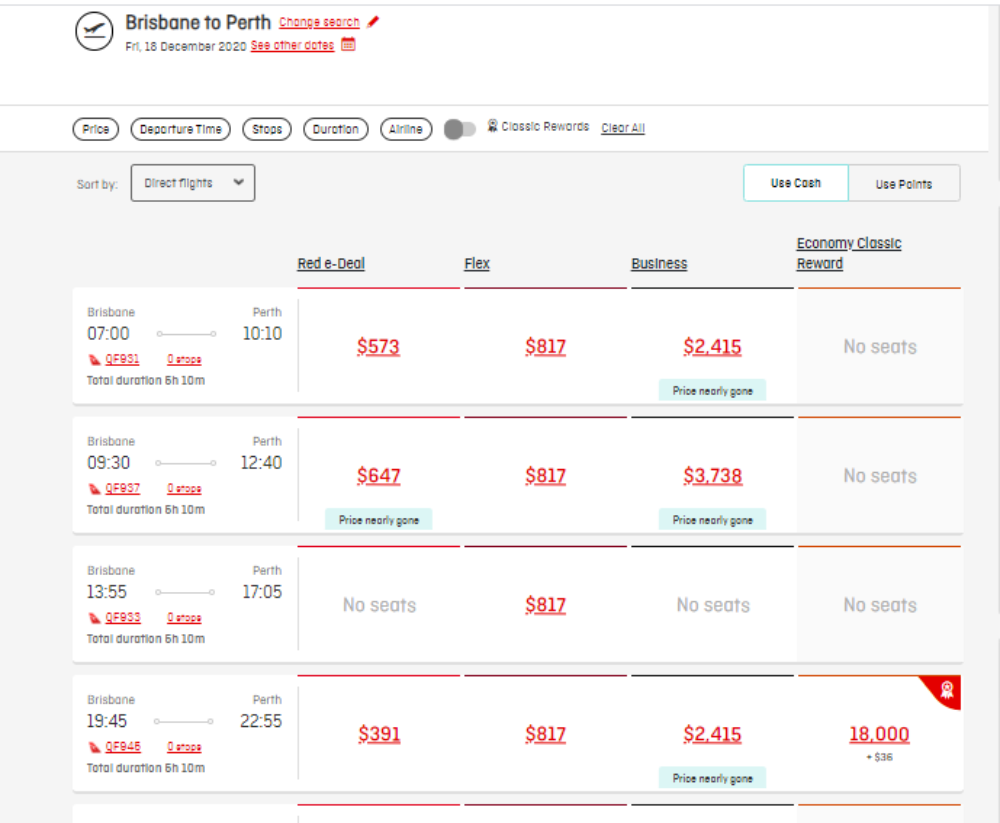The image displays a comprehensive search results screen for flights from Brisbane to Perth. It includes sections for altering the search parameters, which are bordered in red and contain key terms like "Change Search" and "Price." Various flight details are listed in a tabular format, including departure times, airline options, and class types (Coach, Business, Economy). Prices for flights are shown, with amounts ranging from $573 to $18,000, indicating different levels of service and flexibility. The screen features a predominantly white background with some sections bordered in black, and text in both red and black. A notable feature of the layout is the presence of circles, either white or black, which may indicate selection or highlighting of specific options. Flight times and durations are displayed, such as "9:30 to 12:40" and "19:45 to 22:55," along with indicators for availability, with phrases like "No seats."